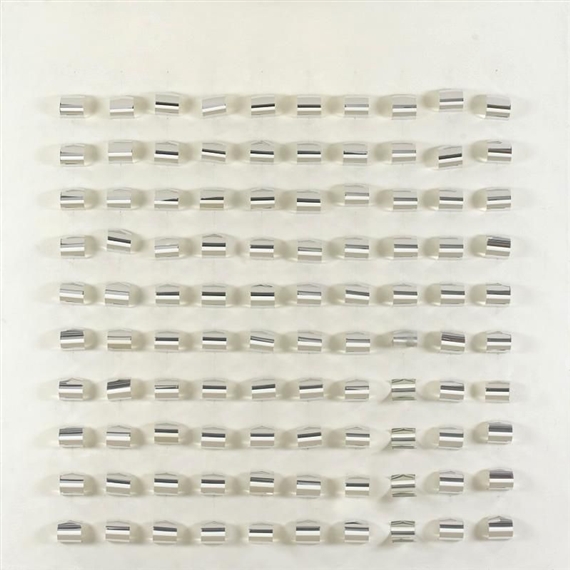The image depicts a color photograph featuring a grid of 100 small, silver, metal cylinder-like objects arranged in 10 rows and 10 columns on an off-white background. Each object resembles a bullet casing without its tip, with alternating black and white stripes adorning their sides. Some of the objects are slightly askew within their rows, adding a touch of irregularity to the otherwise orderly grid. Shadows are present, indicating artificial illumination from multiple directions: shadows from objects on the left side of the image are cast to the right, while shadows from those on the right are cast to the left. The composition includes a larger gap between the top of the image and the first row compared to the gap between the last row and the bottom of the image.